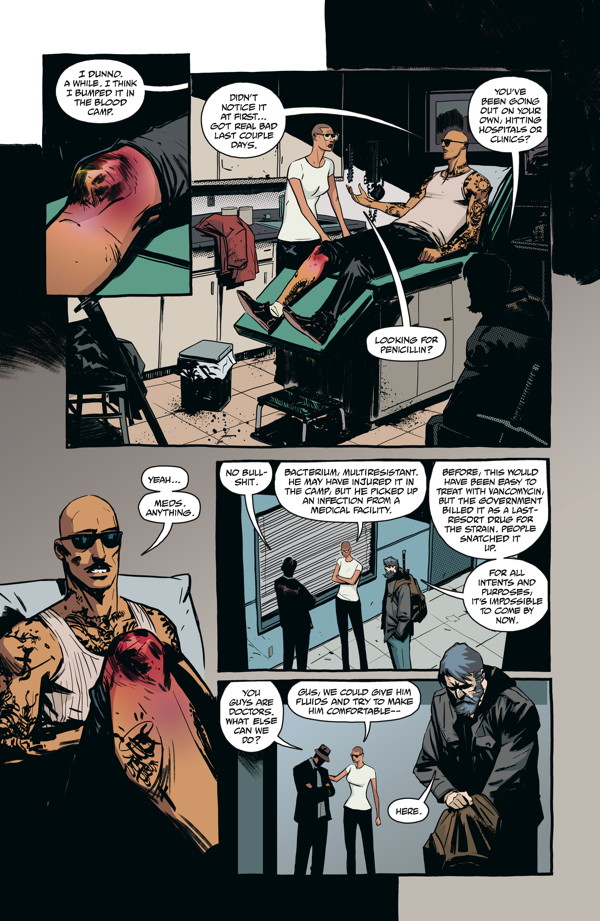The image depicts a page from a colored graphic novel featuring five distinct scenes. At the top left, a vertical black panel shows the dialogue, "I don't know for a while, I think I bumped it in the blood camp," alongside a drawing of a swollen, bruised knee. To the right, a makeshift kitchen-like setting with a makeshift operating table is seen, where a tattooed man in a white tank top, wearing dark sunglasses, lies with his pant leg rolled up, revealing his injured knee.

In the following frame, a close-up captures the same man talking, his speech bubble reading, "Don't notice it at first, it got real bad the last couple of days. You've been going out on your own, hitting hospitals or clinics, looking for penicillin." Below this, two frames depict interactions outside on the street: the injured man and two other individuals, one of whom is a woman also wearing glasses, engage in a conversation.

Overall, the page showcases a sequence detailing the man’s injury and his interactions with others as they discuss his condition and search for medical supplies.